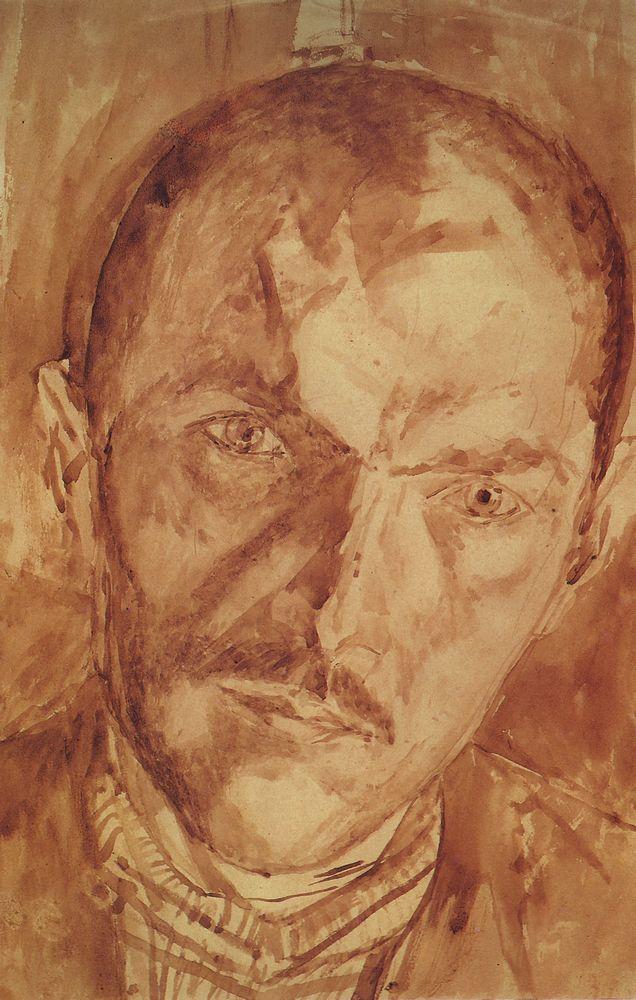This sepia-toned drawing is a semi-realistic portrait of a man, capturing his face down to just below his neck. The man has very short dark hair, possibly balding, with piercing light-colored eyes that contrast with the predominantly brown tones of the artwork. He wears a dark, thin mustache above his closed, thin lips and has a long, sharp nose. His face appears somewhat triangular, framed by heavy dark eyebrows that contribute to his pensive, thoughtful expression. His head is slightly tilted to his left, our right, as he gazes intently into the distance. The man is dressed in a dark jacket over a white shirt that has darker line patterns, giving the impression of multiple layers, possibly including a scarf. His overall demeanor is one of introspection and quiet contemplation.